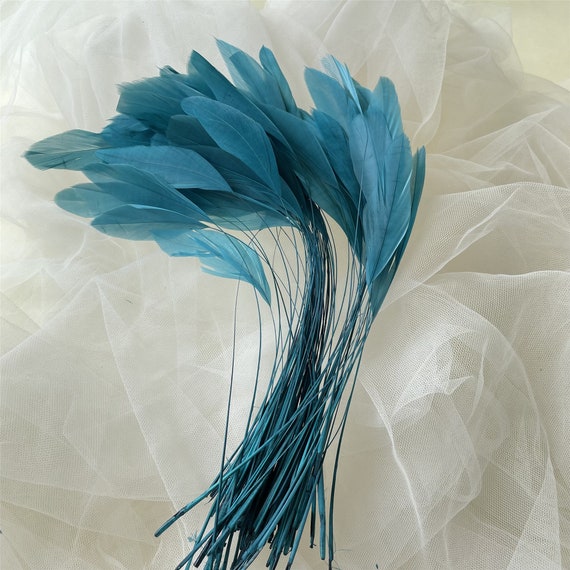The image depicts a meticulously arranged bundle of vibrant blue-teal feathers sprawled across a white, mesh-like, sheer fabric that resembles delicate wedding dress netting. The feathers, appearing somewhat artificial with cheap paper-like stems, possess long, narrow quills that taper to fine points. The collection features over a hundred feathers, each predominantly four to five feet in length. The entire background is dominated by this textured, fluffy netting, creating a somewhat simplistic, 90s-era artwork vibe reminiscent of décor in a doctor's office. The overall scene exudes a sense of minimalistic elegance, evoking the aesthetic of vintage artwork.